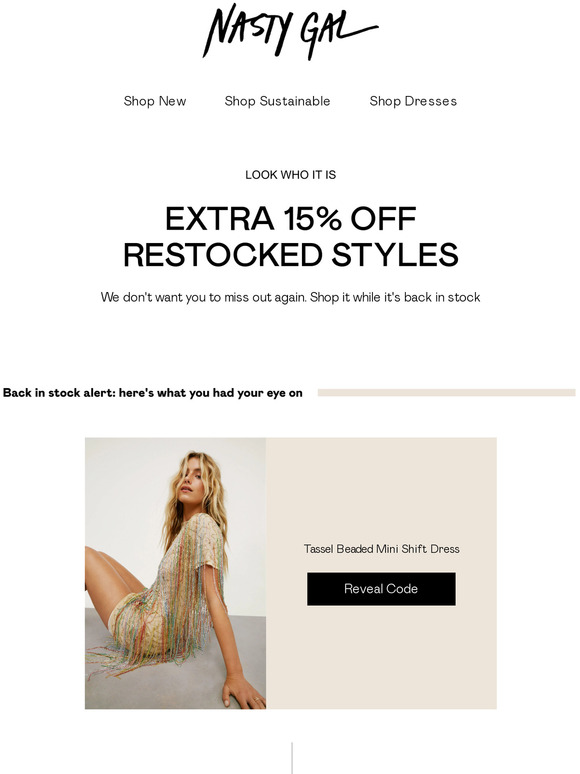The image appears to be from a clothing retailer website, specifically Nasty Gal. The background is completely white, giving it a clean and minimalist appearance. At the top center of the image, "Nasty Gal" is displayed in black, indicating the brand name and logo. Below this, also centered, there are three clickable options: "Shop New," "Shop Sustainable," and "Shop Dresses." 

Further down, the text "Look Who It Is" is prominently displayed. Beneath it, in bold letters, the image announces, "Extra 15% Off Restocked Styles." Accompanying this announcement, smaller text reads, "We Don't Want You To Miss Out Again. Shop It While It's Back In Stock." The bold text "Back In Stock Alert" precedes the phrase, "Here's What You Had Your Eye On."

On the left side of the image is a picture of a model sitting down, showcasing a colorful dress adorned with tassels. The dress is short, highlighting much of the model's legs. The model is blonde, adding to the visual appeal of the presentation.

On the right side, the dress is named "Tassel-Beaded Mini-Shift Dress." Beneath the name, a black horizontal bar contains the text "Reveal Code" in white. The background behind this section is light gray, with the text in black. This minimalist page focuses solely on promoting the "Tassel-Beaded Mini-Shift Dress" from Nasty Gal.